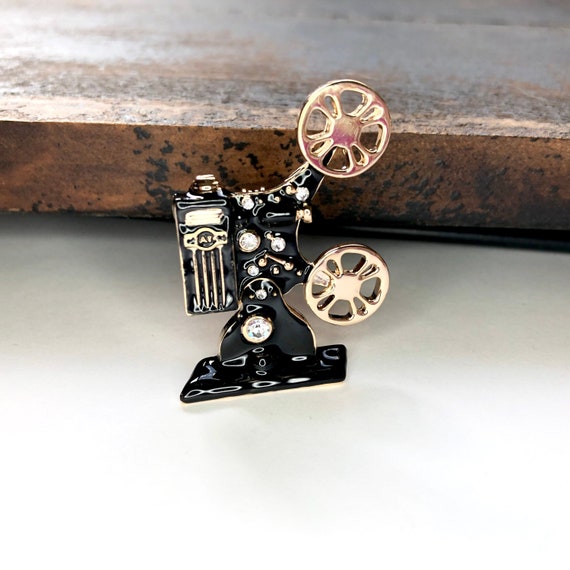The image depicts a highly detailed, decorative figurine designed to resemble an old-time movie projector. The figurine is predominantly painted in a glossy black enamel with gold accents. Key features include two gold movie reel wheels, with one reel displaying a hint of magenta. The projector is adorned with round buttons made from clear gemstones encircled by gold. The front of the figurine has a gold area that appears to bear the initials "AV." The entire piece is set on a white surface, with a background featuring a 3D-textured, rusted metal wall in shades of gray and brown. The figurine stands out due to its reflective surface and meticulous design, offering a nostalgic nod to vintage cinema.